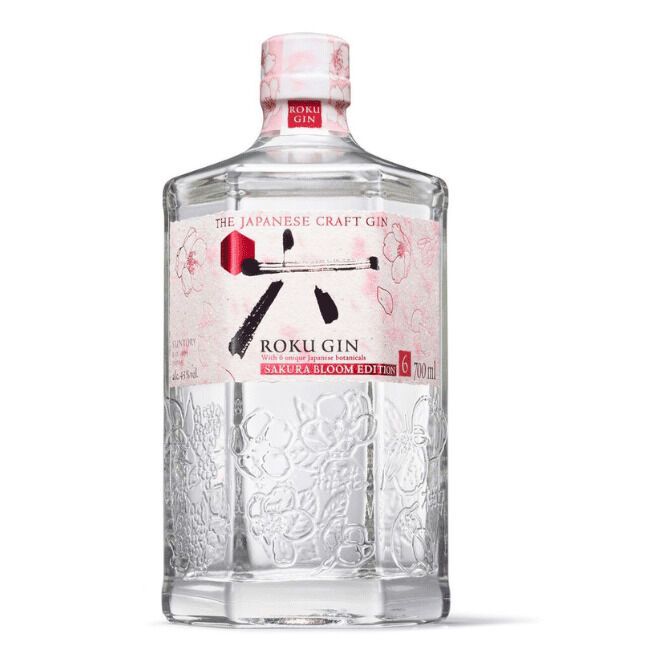The image displays an elegant, decorative bottle of gin known as the Japanese Craft Gin Roku Gin Sakura Bloom Edition. The bottle features a distinctive hexagonal shape with intricate floral designs, possibly Japanese cherry blossom petals, etched into the glass. The label, wrapped around the center of the bottle, is soft rose pink adorned with delicate rose drawings and Japanese characters. It prominently highlights "Japanese Craft Gin" at the top, with "Roku Gin" and "Sakura Bloom Edition" accentuated in white on a darker pink background, and it mentions "six unique Japanese botanicals" and the volume "700 milliliters." The cap is a combination of pink and white, with a red square label that reads "Roku Gin" in white text. The bottle appears to be full and sealed, suggesting its contents remain intact.